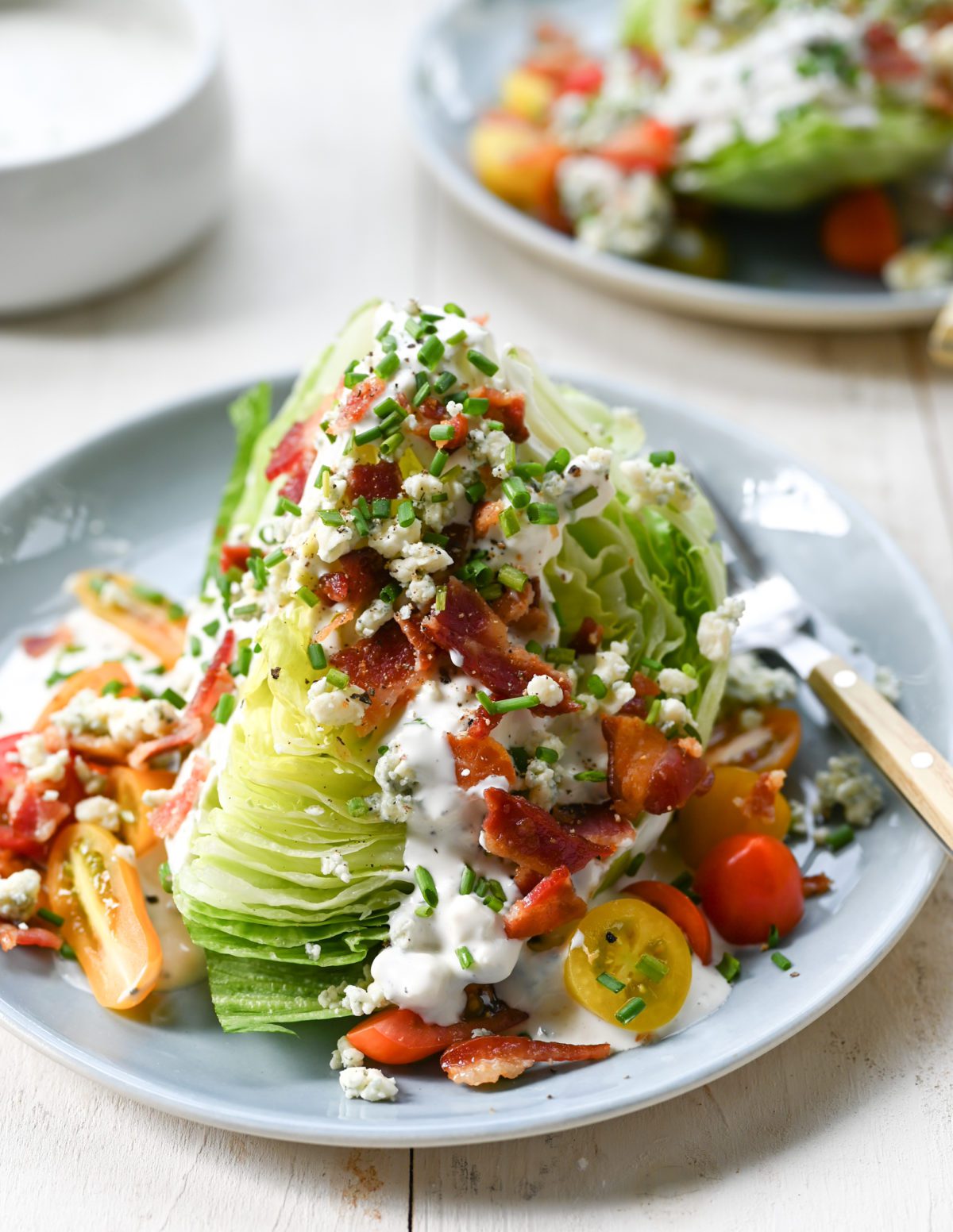The full-color photograph, taken indoors and professionally staged, depicts a vertical, borderless image focusing on a complex, vibrant salad in the foreground. The background, primarily a white wooden table, features subtle light in the upper-left corner. At the center is a white, slightly concave plate, partially cut off on the left side of the image, showcasing an elaborate wedge salad. The salad, composed of a mound of lettuce layers, is adorned with a mix of toppings including bacon bits, crumbled blue cheese, and dressing. Interspersed within are colorful elements like orange slices, red and white pieces suggestive of tomatoes or cheese, and a cherry tomato positioned near the bottom right. A fork rests on the plate, extending out of the right edge of the image. In the upper portions of the frame, there's a plain white bowl on the left and a blurred plate with another salad on the right, partially out of the frame.